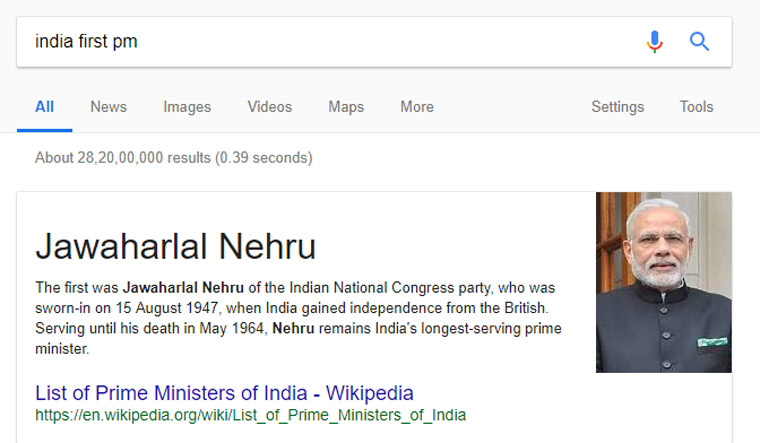### Detailed Image Caption:

The image displays a search engine window with a white background. At the very top of the window, there is an elongated search bar containing the text "India first PM or prime minister." Below this search bar, an eight-option navigation menu is visible. The first option, "All," is selected and is followed by "News," "Images," "Videos," "Maps," "More," "Settings," and "Tools."

Directly beneath the navigation bar, the search engine displays the text "About 28,200,000 results in 0.39 seconds." The main body of the window focuses on the search query. At the top, in large black text, the search results prominently display the name "Jawaharlal Nehru."

Further detailed information follows, beginning with the text: "The first Prime Minister of India was Jawaharlal Nehru of the Indian National Congress Party, who was sworn in on August 5th, 1947, when India gained independence." Below this description, a blue hyperlinked text reads "List of prime ministers of India - Wikipedia," with the corresponding green URL displayed below it.

To the right of this textual information, there is a color portrait photo of Jawaharlal Nehru. Nehru is depicted wearing a gray or light black buttoned-up jacket with a high collar. He is also wearing glasses, with a white beard and white hair.